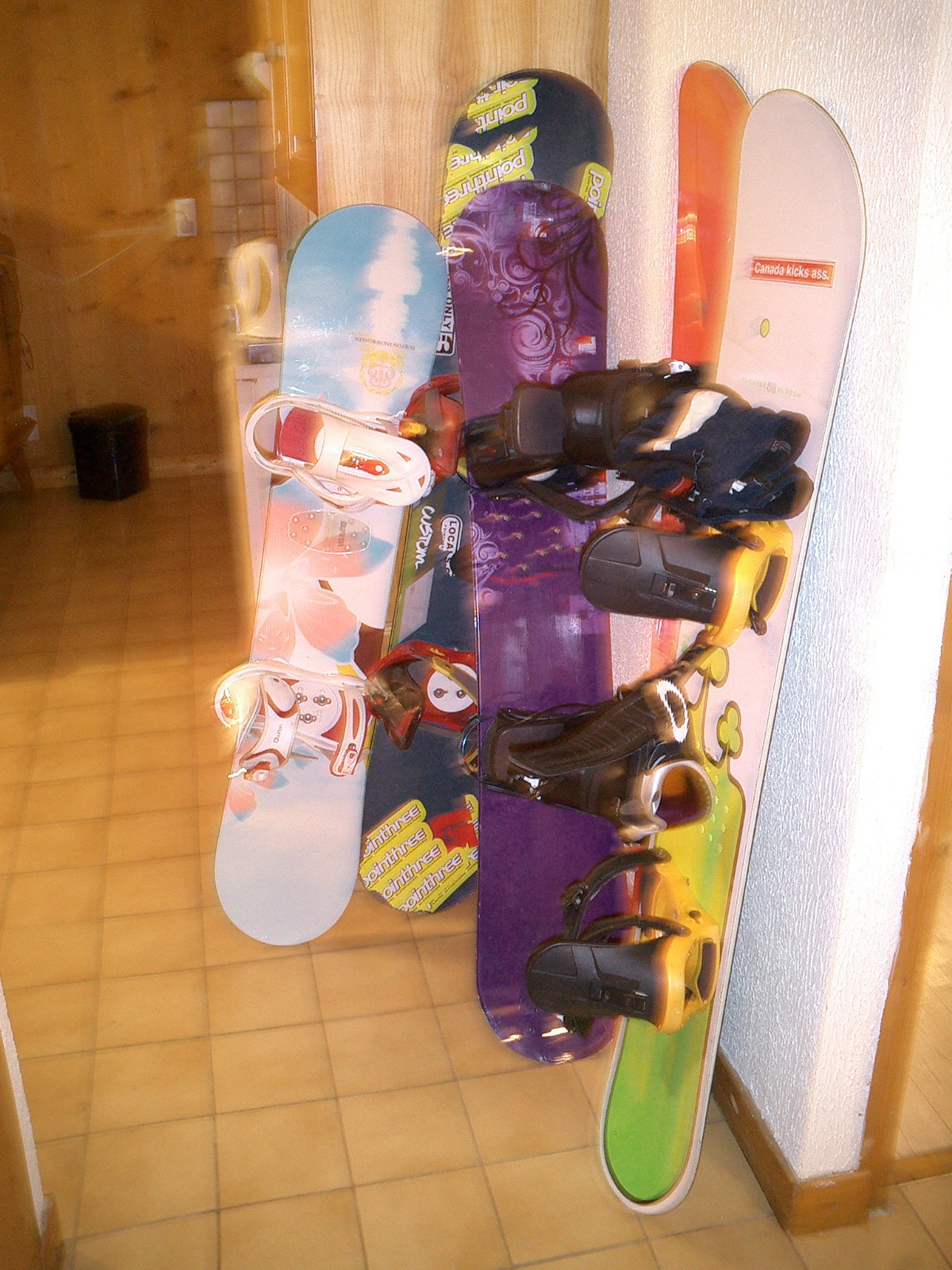This photograph captures a collection of five distinct snowboards resting against a white textured wall with wood baseboards in a household setting, likely a hallway or kitchen corridor. The aspect emphasizes tan or beige tiles on the floor and wooden cabinetry, with additional elements such as a small black trash can and possibly laundry equipment, including a detergent bottle and the corner of a washing machine, suggesting a multi-use space.

The snowboards vary in size and design, featuring eye-catching colors and patterns. The closest snowboard is primarily green and yellow with a white upper section that displays the phrase "Canada Kicks Ass." A pair of gloves is draped over its footrest. Next to it, an orange snowboard, while adjacent to it, a purple snowboard showcases abstract designs. Further along the row is a predominantly blue snowboard with yellow and white logos, though the text is not fully legible. The fifth appears blue and white as well. Additional background details include a wooden kitchen cabinet and a countertop holding what seems to be a white pitcher or electric tea kettle.